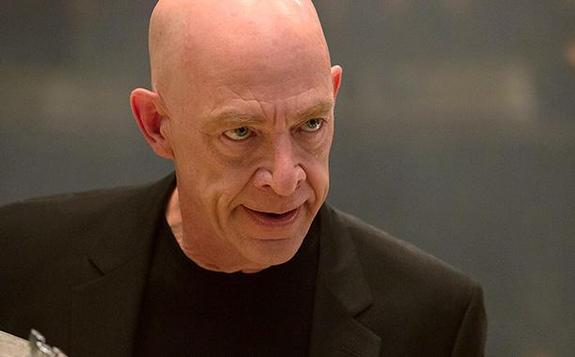This is a detailed, full-color photograph of JK Simmons, an older white male with a bald head, clean-shaven face, and light-colored eyebrows. He is wearing a black t-shirt under a black blazer. His intense, serious expression suggests a combination of anger and disappointment, reminiscent of his character as a harsh music professor in the film "Whiplash." He appears to be speaking, with his mouth open and lips forming words, while his gray or blue eyes are directed slightly to his left. The background is blurred and predominantly gray, with an indistinct white and silver object visible in the right corner.